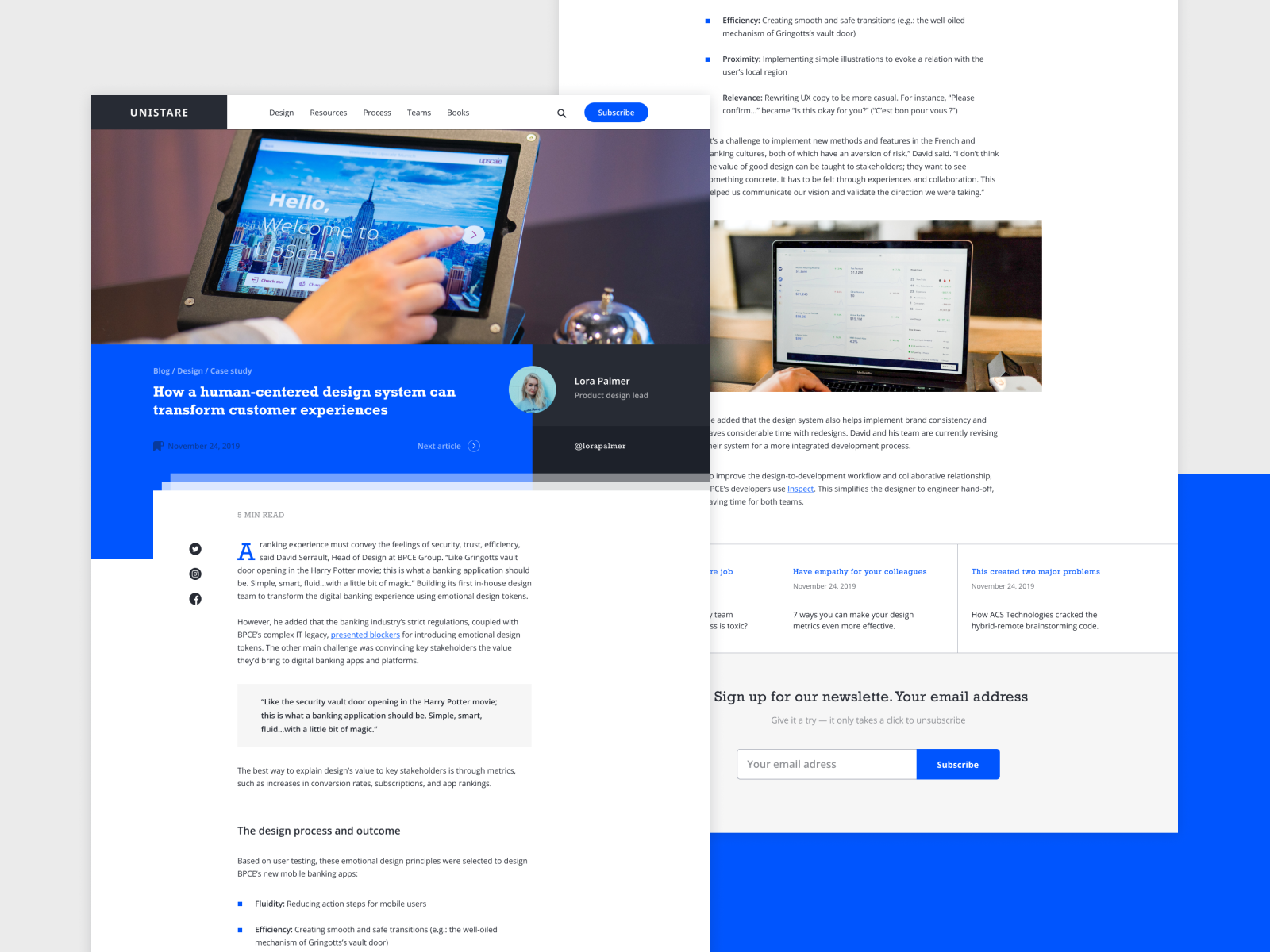In the image, the upper left-hand corner features a banner labeled "Unistair." Adjacent to this banner is a white navigation bar containing various clickable tabs, followed by a search bar. Below this is a blue banner with illegible text at its center. As we move further down the image, we see a close-up of a Caucasian male hand poised over a laptop, seemingly ready to click on a white arrow located on the right side of the screen. The laptop display shows a homepage with the partially visible greeting "Hello, welcome to," though the remainder of the text is indiscernible. Beneath this section, there is a prominent blue banner with the title "How a human-centered design system can transform customer experiences." To the left of this text is a circular profile picture of a Caucasian female named Laura Palmer. Below this banner, the screen is filled with a substantial block of text. On the left side of the white background, there are social media icons for Twitter, Pinterest, and Facebook.